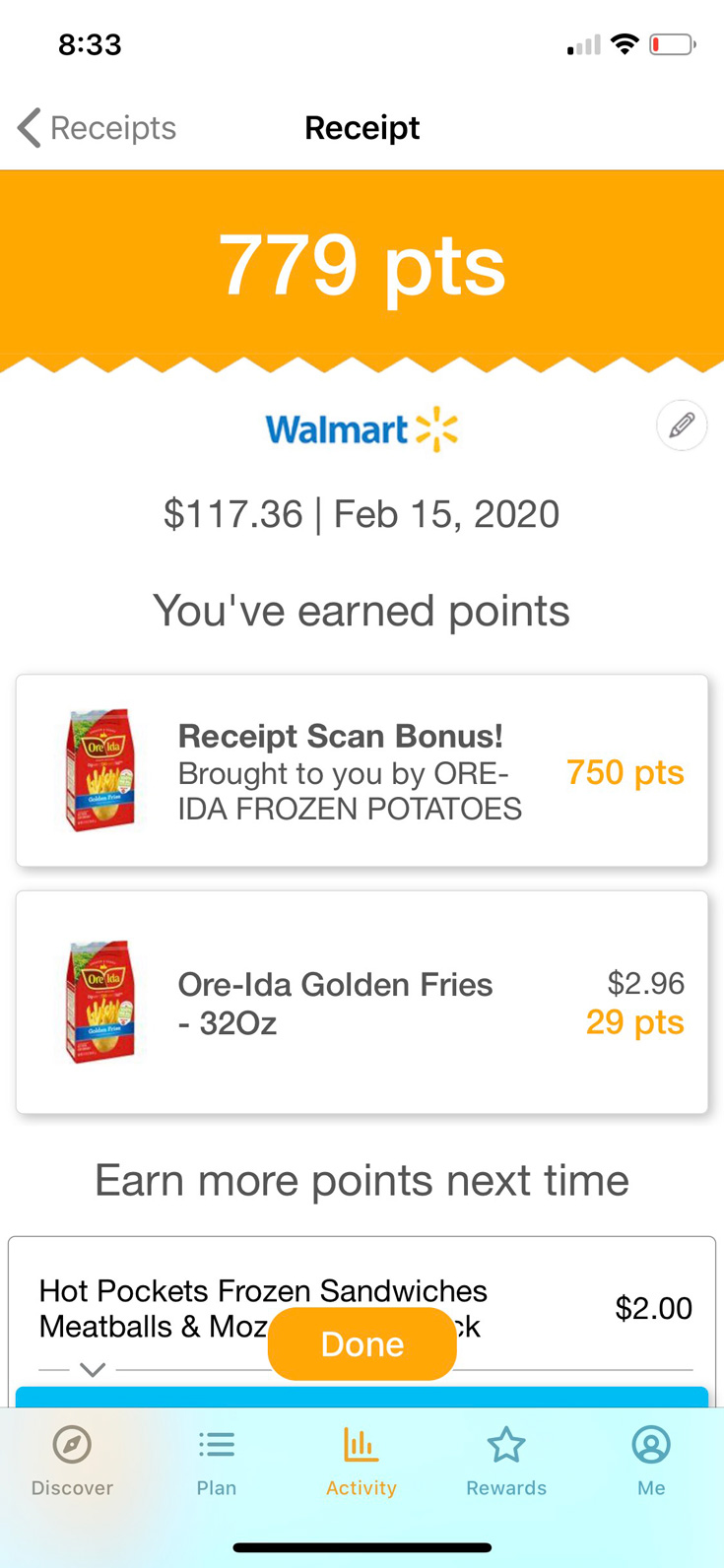The screenshot displays a cell phone interface at 8:33 AM, shown at the top bar. On the right, the phone has only one bar of signal strength, is connected to Wi-Fi, and displays a nearly depleted battery with a red line. The main heading is "Receipt," with "Receipts" in grey and a left arrow, and "Receipt" centrally positioned in bold black text. 

Beneath this, a yellow banner with white text indicates "779 PTS" or "779 points," with a distinctive scalloped bottom edge. Below the banner, the Walmart logo is visible, next to a pencil icon symbolizing the option to edit. The amount "$117.36" is displayed prominently, followed by a vertical line separating the purchase date, "February 15, 2020." The text "You've Earned Points" appears below in black.

The screen features two rectangular sections highlighting earned points. The first rectangle, titled "Receipt Scan Bonus brought to you by Ore-Ida Frozen Potatoes," awards 750 points. The second rectangle details "Ore-Ida Golden Fries, 32 ounces, $2.96," worth 29 points. To the left of these entries, an image of the product—a red bag with french fries—is shown.

Underneath these details, the text "Earn More Points Next Time" is displayed. Further down, "Hot Pocket Frozen Sandwiches, $2" is noted. The bottom navigation menu includes options: "Discover," "Plan," "Activity," "Rewards," and "Me."